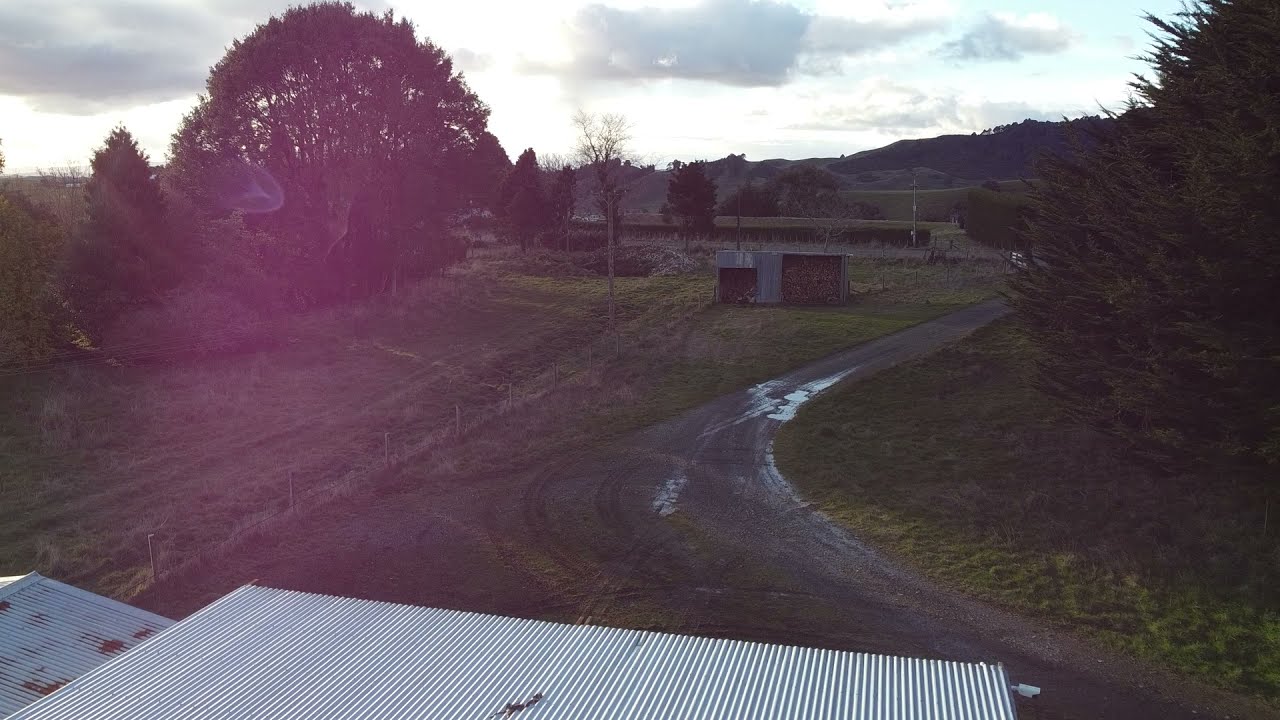The image depicts a rustic countryside scene, captured from an elevated vantage point, possibly a roof. Dominating the foreground are two tin roofs—one belonging to a larger structure and the other to a smaller one, both exhibiting rust. The structures appear rundown, with the shed showing visible signs of disrepair, including exposed plywood and missing doors. Stretching from the bottom right and meandering towards the center before veering off to the top right is a wet, gravel or dirt road, marked with puddles, indicating recent rain.

Flanking this road are grassy areas, showcasing shades of brown and green, with additional greenery from trees positioned on both sides: larger trees are on the left, while a single prominent tree stands on the right. These trees have lush green leaves. In the middle distance, there is an old shed, slightly off-center to the right, partially concealed by the surrounding foliage.

Further back, the landscape opens up to gentle, rolling hills dotted with more trees. The sky above is light blue, adorned with fluffy clouds through which the sun attempts to peek, adding a softer light to the scene. The overall ambiance is serene and somewhat melancholic, typical of a countryside home. There is no text present in the image.